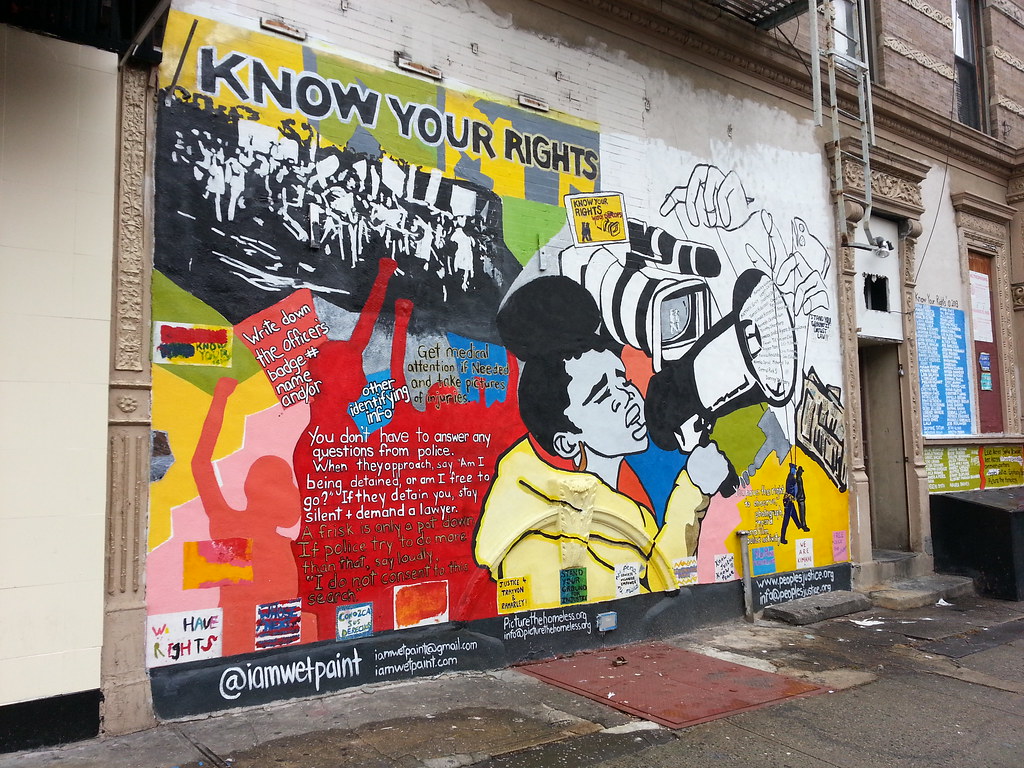The image depicts a vibrant and detailed street art mural on the wall of a city building, characterized by colorful hues including yellow, red, orange, green, and shades of gray, with touches of black and white. Central to the mural is a powerful scene of a woman with her hair tied in a bun, wearing a yellow jacket, passionately speaking into a megaphone. Behind her, a figure is recording with a video camera, and the scene extends to show a group of people gathered, potentially at a protest. Another striking feature includes puppeteer-like fingers manipulating two police officer figurines with strings, emphasizing themes of control and authority.

Across the mural, crucial messages are prominently displayed: "Know Your Rights," "Write down the officer's badge number, name, and other identifying info," "Get medical attention if needed and take pictures of injuries," and "You don't have to answer any questions from police. When they approach you, ask if you are being detained or are free to go; if detained, stay silent and demand a lawyer." The bottom of the mural is signed by the artist with the handle "@iamwhatpaint."

This artwork not only captures a moment of activism but also serves as an educative piece, underscoring the rights of individuals in encounters with law enforcement.